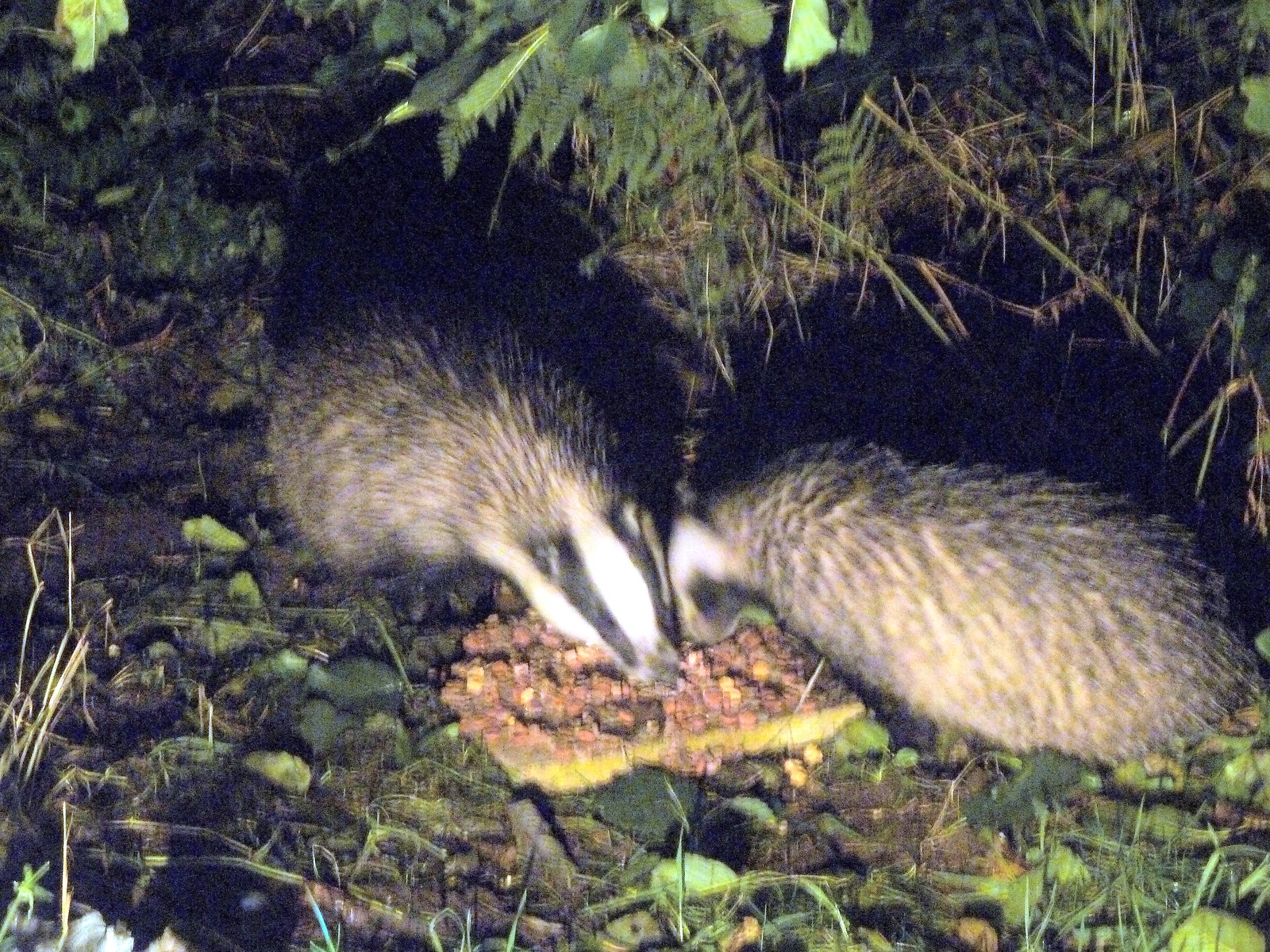In this blurry and noisy nighttime image, two animals are captured outdoors, seemingly in a damp, forested area. The scene reveals mud, green shoots of grass, and various ferns and leaves. The animals appear to have a round shape, which could suggest they are raccoons or ferrets, though their exact species is hard to determine. Their brown fur and distinct black stripes around their eyes further hint at raccoons. Despite the motion blur, it is clear they are nibbling on some kind of food, possibly a piece of pizza or a fruit with visible seeds. The camera flash highlights the wet ground and the surrounding ditch area, adding to the night-time effect of the image.